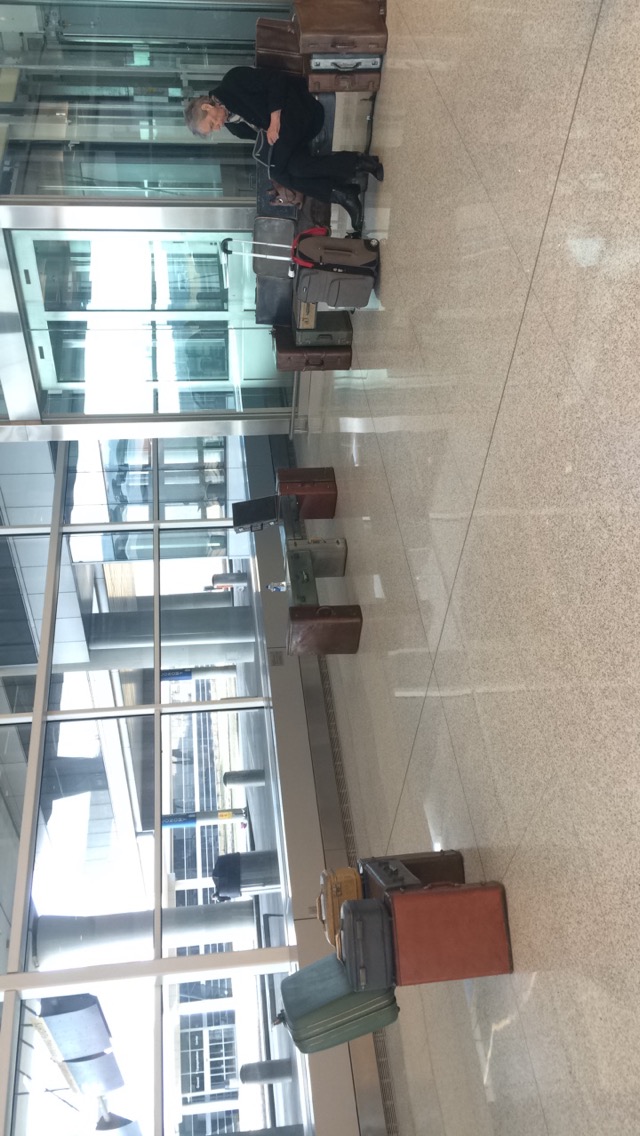The image depicts a unique airport setting with a series of creatively designed benches made from vintage suitcases. Three benches are arranged in a semicircle, each featuring a brown seat, with armrests and backrests fashioned from suitcases. Behind the benches are large glass panels, which offer a view of another section of the airport also lined with glass panels. On the far right bench, an older man with short gray hair, dressed entirely in black including a black overcoat and black dress shoes, sits cross-legged. He is absorbed in reading a book, with his gray suitcase positioned in front of him and its steel handle extended. The flooring of the airport consists of shiny, tan khaki tiles, contributing to the overall modern aesthetic. The setting overlooks a pickup roadway, with a covered walkway visible in the background. The scene captures a quiet moment of travel, juxtaposed against the hustle and bustle of airport activities.